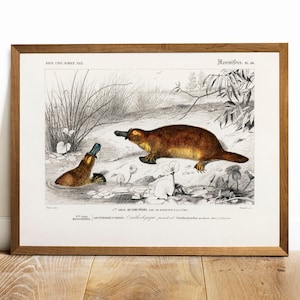This image, framed in a thin oak frame, sits against a wall on an oak plank floor. The artwork, resembling an Audubon style illustration, features two hand-drawn platypuses with subtle coloration set against a beige to white background. The scene, a wintry landscape under a gray sky, juxtaposes the colored animals with the monochromatic surroundings. On the lower left, one platypus emerges from a pond up to its waist, focusing on the other platypus on the rustic, snowy shore. The shore, a mix of rocky terrain and dying weeds, is meticulously sketched in black ink. The animals exhibit detailed coloring: dark brown on their upper bodies, tan on their bellies, and gray on their snouts. Additionally, a black sketch of plant growth decorates the bottom right corner. Above the illustration, a tiny title and the artist’s signature are inscribed in the white space, enhancing the authenticity and artistic value of this carefully framed piece.